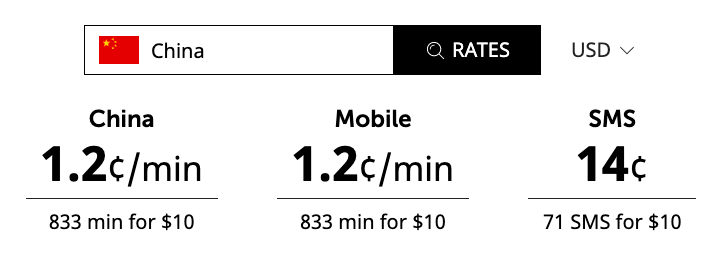The website features a minimalist design with a predominantly white background. On the left side, there is a white box containing the word "China" alongside an icon resembling the Chinese flag—a red background with a large gold star and smaller gold stars. Adjacent to this box, a black section features the word "Rates" and a search icon. To the right of this, it says "USD" with a downward-facing arrow.

Below this header, the word "China" appears prominently in large, bold letters. Underneath, the text reads "1.2 cents/min" followed by a line indicating "833 minutes for $10." Next to this information, the word "Mobile" is displayed along with the same rate of "1.2 cents/min" and the same allowance of "833 minutes for $10." Adjacent to this is the word "SMS" in bold black text, stating a rate of "14 cents" per message, followed by "71 SMS for $10" beneath a separating line.

The website lacks additional context or a clear header to explain the purpose or origin of these rates, suggesting it is a straightforward listing of telecommunication costs without further elaboration.